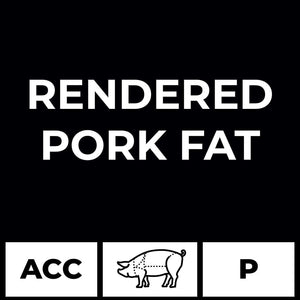This digital poster is a square-shaped black and white design. Centrally positioned at the top, white capitalized sans-serif text reads "RENDERED" on the first line and "PORK FAT" on the second line, both centered. Near the bottom fifth of the image, three horizontal white rectangles are aligned in a row. The leftmost rectangle features the black capital letters "ACC." The middle rectangle displays a black line drawing of a pig seen from the side, with dotted lines indicating different meat cuts. The rightmost rectangle contains a single black capital letter "P." The rest of the background is solid black, creating a stark contrast with the white elements.